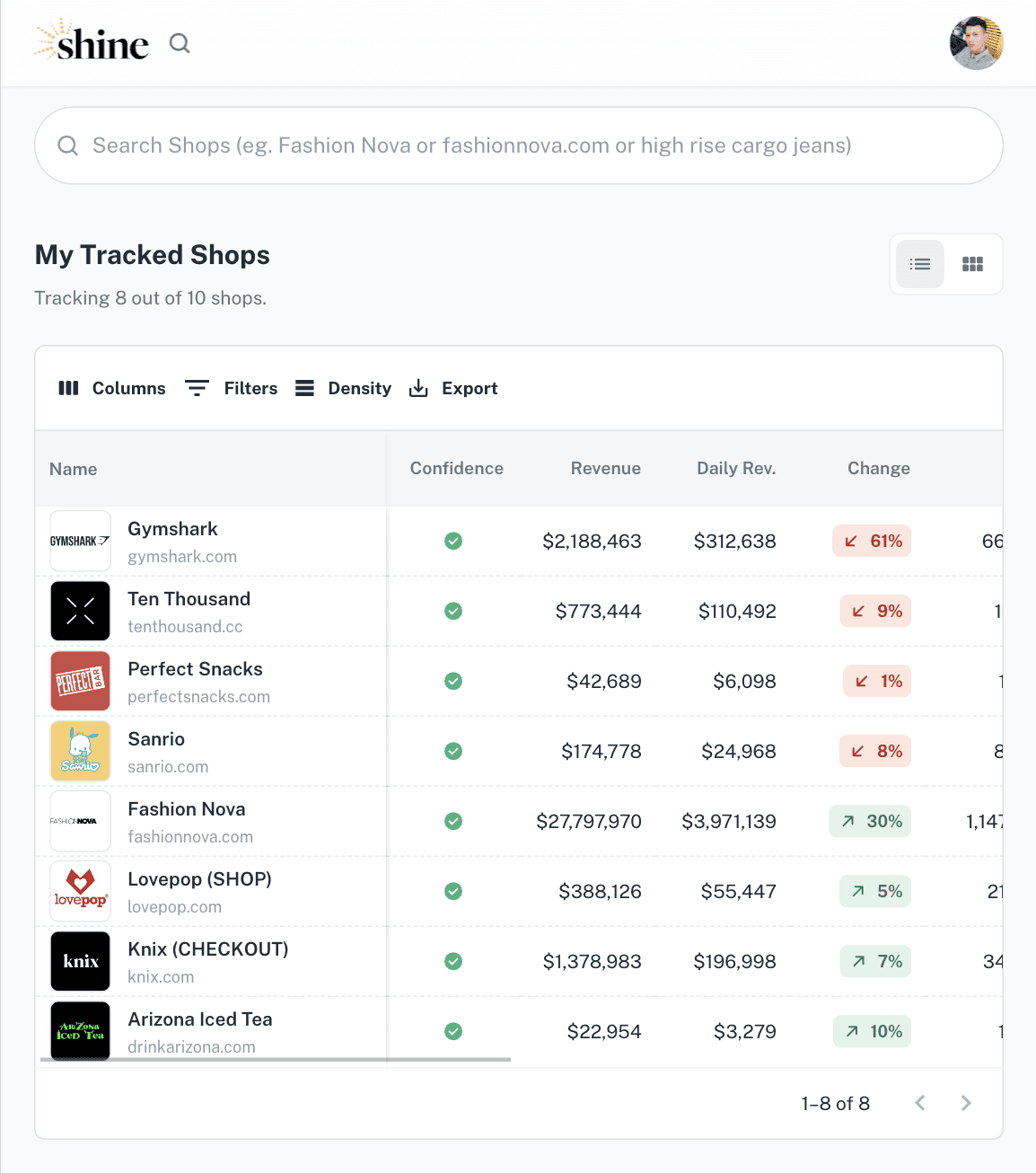The image depicts a web page layout for a site named "Shine," prominently featuring its logo resembling a radiant sun positioned adjacent to the site's name. Beneath the header, there is a search bar labeled "Search Shops," encouraging users to input terms such as "Fashion Nova," "fashionnova.com," or "High Rise Cargo Jeans." Directly below the search bar is a section titled "My Tracked Shops," indicating that 8 out of a possible 10 shops are currently being tracked.

Further down, the interface presents a set of tools and options including columns, filters, density, and export functionalities. Following these tools, the page lists several shops with their respective logos and names in a tabular format. The listed shops, in order, include Gymshark, 10,000, Perfect Snacks, Sanrio, Fashion Nova, Love Pop, Nick's, and Arizona Ice Tea.

Each shop entry is accompanied by several metrics, suggesting that the page is designed to track the business performance of these shops. The metrics displayed include a Confidence Rating, Revenue, Daily Revenue, and Change, providing a comprehensive overview of each shop's financial status and performance trends.